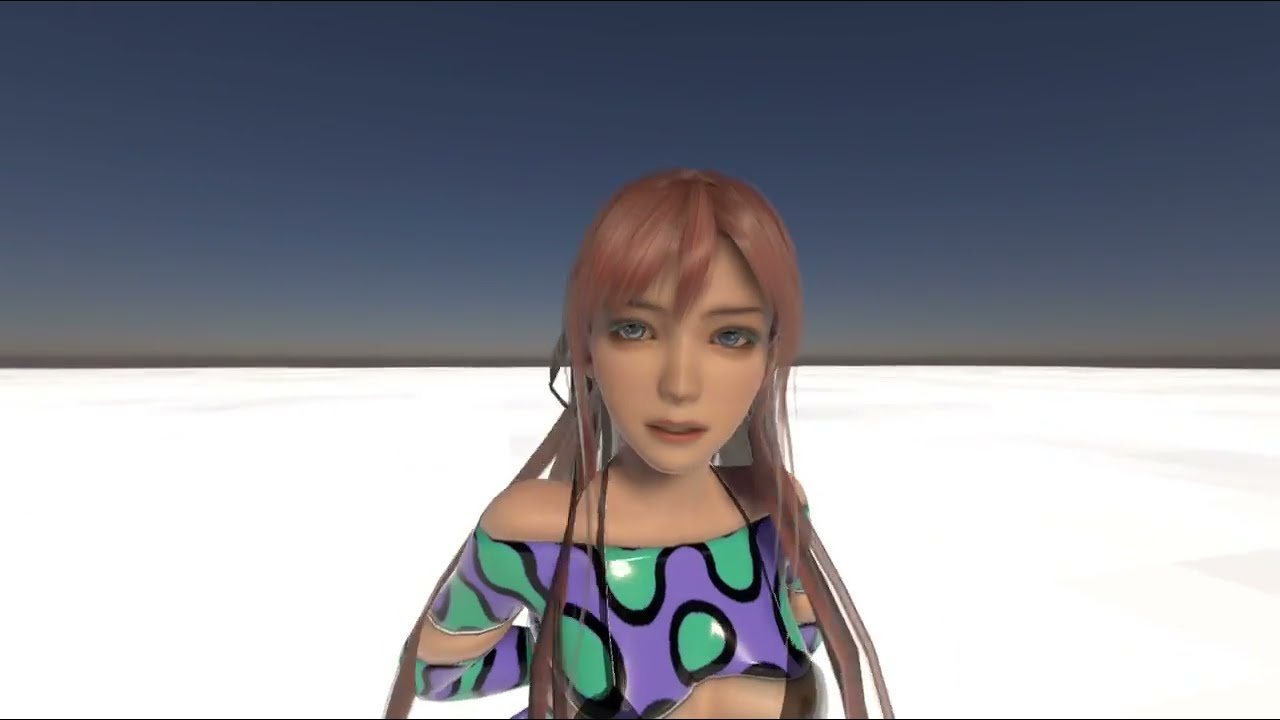The image is a detailed digital rendering of a woman positioned in the center, looking directly at the camera. She has long, reddish-brown hair that flows past her shoulders and has a light skin complexion. She is wearing a distinctive lime and purple shirt featuring a splatter pattern with black accents along the design. The shirt is cut off at her shoulders, revealing some bare skin and potentially exposing her midriff. The background is minimalistic, with a white surface suggesting an outdoor setting, while the upper part of the backdrop transitions into shades of blue and gray, devoid of clouds. The overall scene is brightly lit, giving a clear and vivid appearance. There are no other objects or text in the image, making the woman the sole focus of the composition.